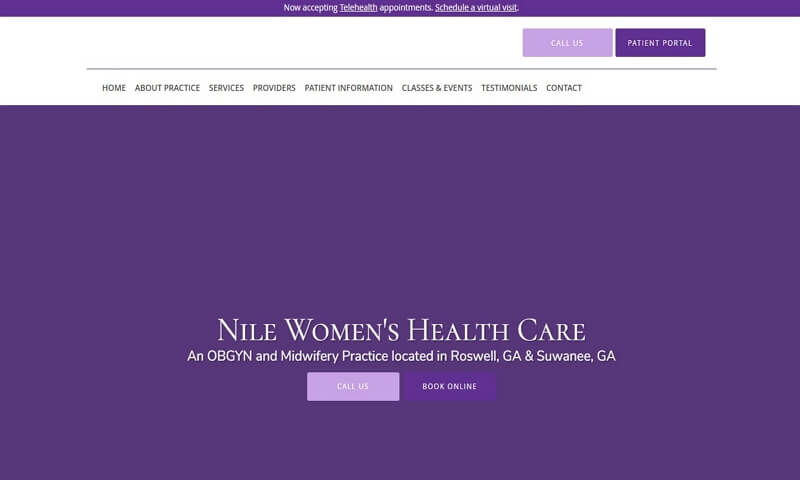The top section of the image features a thin purple border with a white center that reads, "Now Accepting Telehealth Appointments Per Your Schedule, A Virtual Visit," with the last line underlined in white. 

On the right side, two rectangular boxes can be seen. The first box, which is light purple and white, says "Call Us." The second box, in regular purple and white, reads "Patient Portal."

A thin black line runs horizontally across the page. Below this line are various tabs, all in black text. From left to right, they read: Home, About Practice, Services, Providers, Patient Information, Classes & Events, Testimonials, and Contact.

The rest of the page features a solid purple background, the same shade of purple as the top border and one of the rectangles mentioned earlier. Towards the bottom, another white rectangle contains the title "Women's Healthcare" with each word capitalized. 

Underneath, it specifies, "OBGYN and Midwifery Practice located in Roswell, GA and Suwanee, GA," with each location capitalized and followed by a comma.

At the bottom of the page, there are two purple boxes. The first box says "Call Us" in white text, and the second box, which also features white text, reads "Book Online," both in all capital letters.